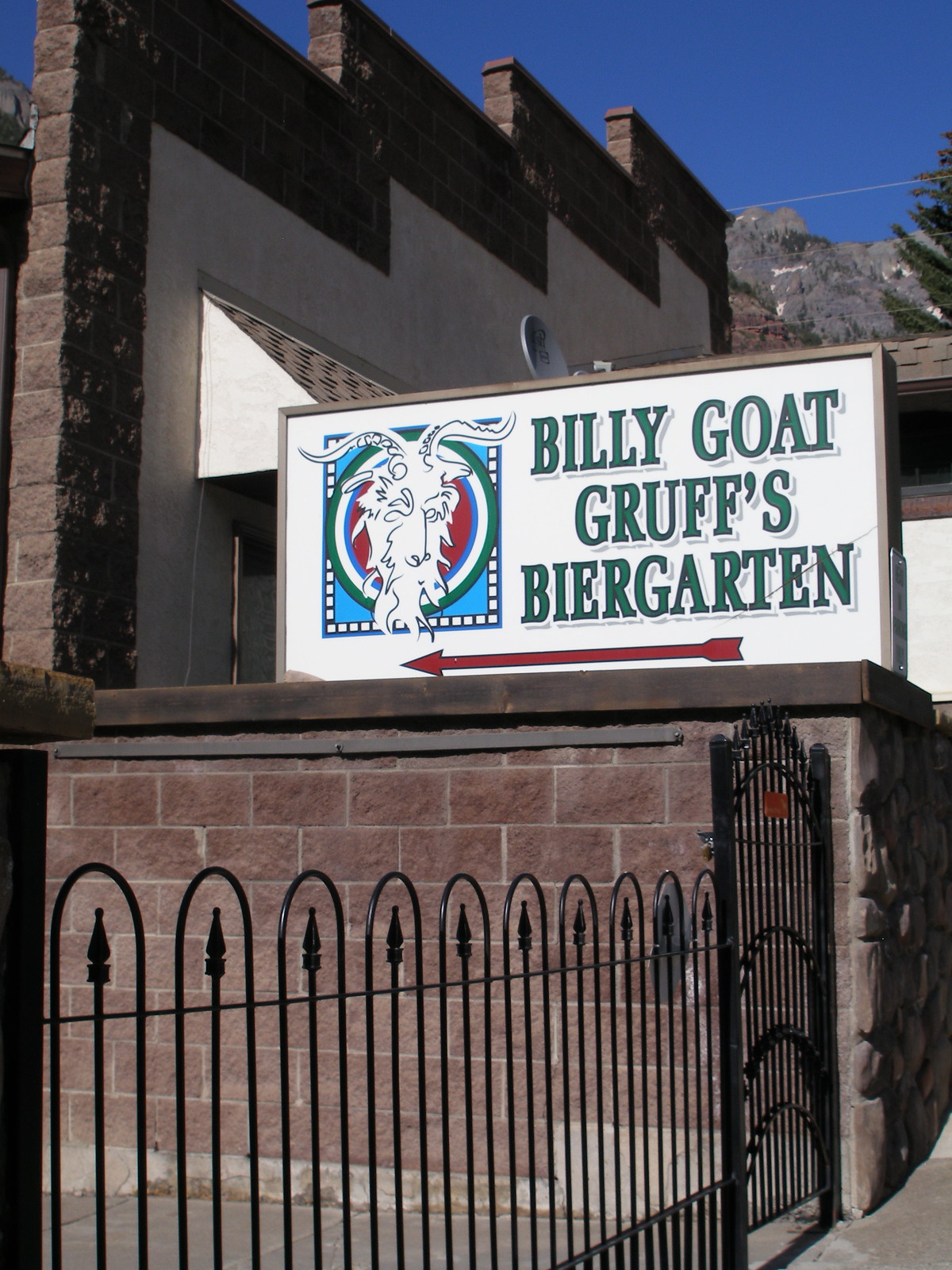This detailed photograph depicts the exterior of Billy Goat Gruff's Beer Garden, framed by a mix of natural and architectural elements. The focal point is a large white sign situated atop a reddish brick half-wall, encased in a metal frame with a brownish-brass hue. The sign itself features a stylized image of a goat's face set within a concentric circular design of red, blue, white, and green outlines. To the right of this logo, bold green letters spell out "Billy Goat Gruff's Beer Garden," with a red arrow pointing left beneath the text. The entire structure is flanked by an ornate black iron gate, which serves as an entryway to the beer garden. In the background, one can make out the rugged peaks of rocky mountains and a crystal-clear blue sky, enhancing the idyllic and inviting atmosphere of the scene.